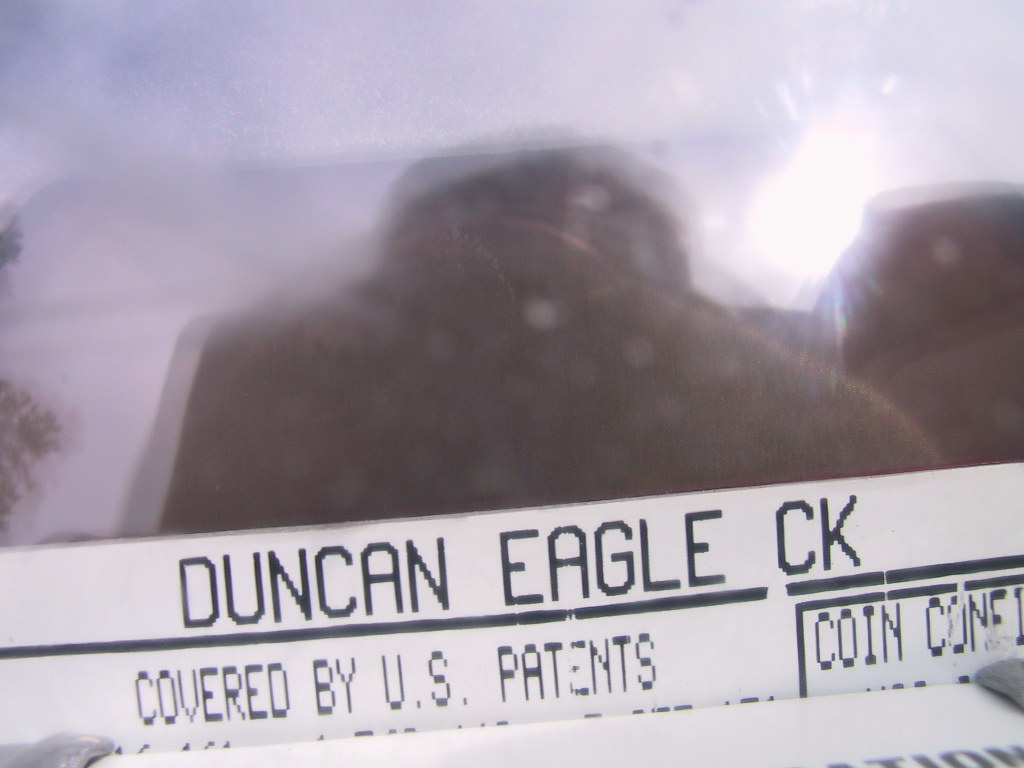This black-and-white photograph presents a surreal landscape dominated by two gigantic rock formations, captured in a somewhat blurred fashion. At the bottom of the image, a large white sign printed with black text reads: "Duncan Eagle CK and covered by U.S. patents and coin cone." The sky above, although grey in the monochrome palette, appears to be bright, with the sun faintly visible behind scattered clouds. On the left side of the frame, part of a tree intrudes into the scene, adding a touch of natural texture. 

The rock formations are the focal points of the photograph. One of these colossal stones rises in a unique shape, reminiscent of a shoulder and neck, culminating in a small, flat area at its peak before gradually curving downwards. Adjacent to it stands another massive rock, together creating a striking geological contrast against what appears to be distant mountains faintly outlined in the background. The overall composition conveys a sense of timeless grandeur and enigmatic beauty.